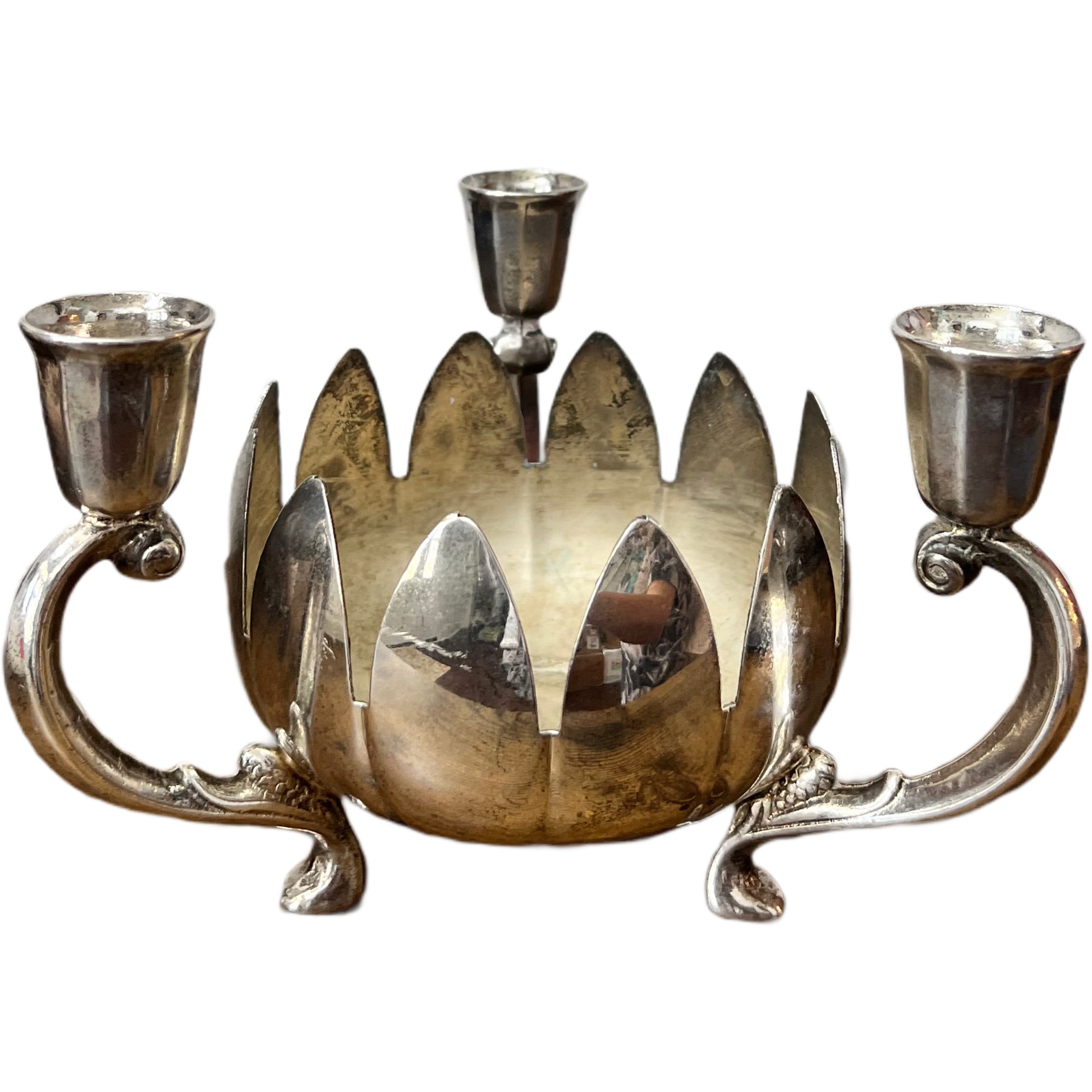The image features a striking silver antique object set against a stark white background, lending it an ethereal appearance. The center of the object resembles an open flower with ten petal-like extensions, each intricately designed and displaying signs of aged polish. The middle forms a bowl that suggests multiple uses, possibly for holding small items or even candles. Supporting this central element are three ornate arms extending outward, each capped with a small cup-like holder that could also accommodate candles. The silver surface is reflective, with visible indentations and rustic designs adding to its antique charm. In the reflection, the arm of someone wearing a patterned shirt is faintly discernible, suggesting a room with two windows and various indistinct objects, possibly cloth or other materials. The overall piece combines elements of both elegance and historical craftsmanship.